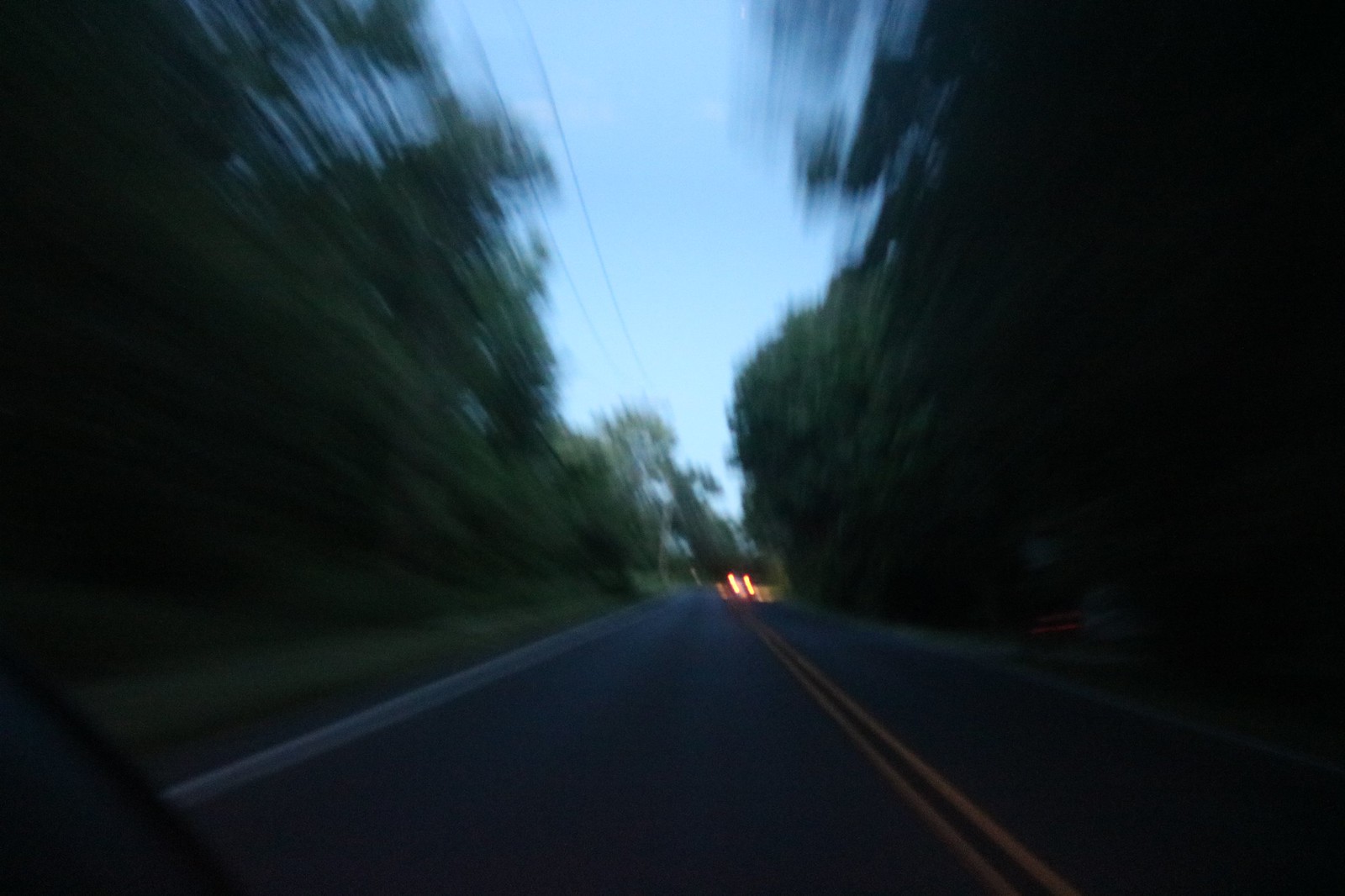A blurred image captures the sensation of motion along a dark paved road with distinct yellow lines marking the separation of opposing traffic lanes. The sides of the frame are flanked by indistinct, blurry shapes that suggest dense trees, reinforcing the impression that the photo was taken at speed. In the distance, faint taillights of a car are just visible, adding depth and a sense of direction to the scene. Above, the sky transitions smoothly from the tree canopy into a serene blue, evoking the feeling of emerging from a forested area into sunlight.